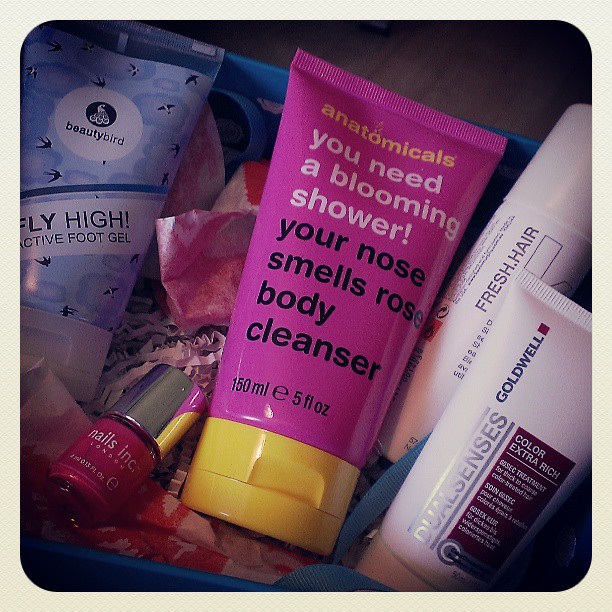The image showcases a curated travel gift basket containing various beauty products, perfect for someone on the go. Housed in a bright blue plastic basket lined with crumpled white tissue paper, the collection features several small-sized items. Dominantly displayed is a vibrant pink bottle with a yellow cap labeled "Anatomicals You Need A Blooming Shower Your Nose Smells Rose Body Cleanser, 150 ml / 5 fluid ounces." To its right, there's a white cylindrical can of hairspray inscribed with “Fresh Hair.” The bottom right contains a bottle of Goldwell Dual Senses Color Extra Rich, likely a shampoo. On the left side, a blue tube labeled "Fly High Protective Foot Gel" is visible. Adjacent to it in the bottom left corner, there's a small vial of red nail polish marked "Nails Inc." The basket's festive appearance is enhanced by decorative shredded paper, making it an appealing and practical kit of health and beauty essentials for a trip.